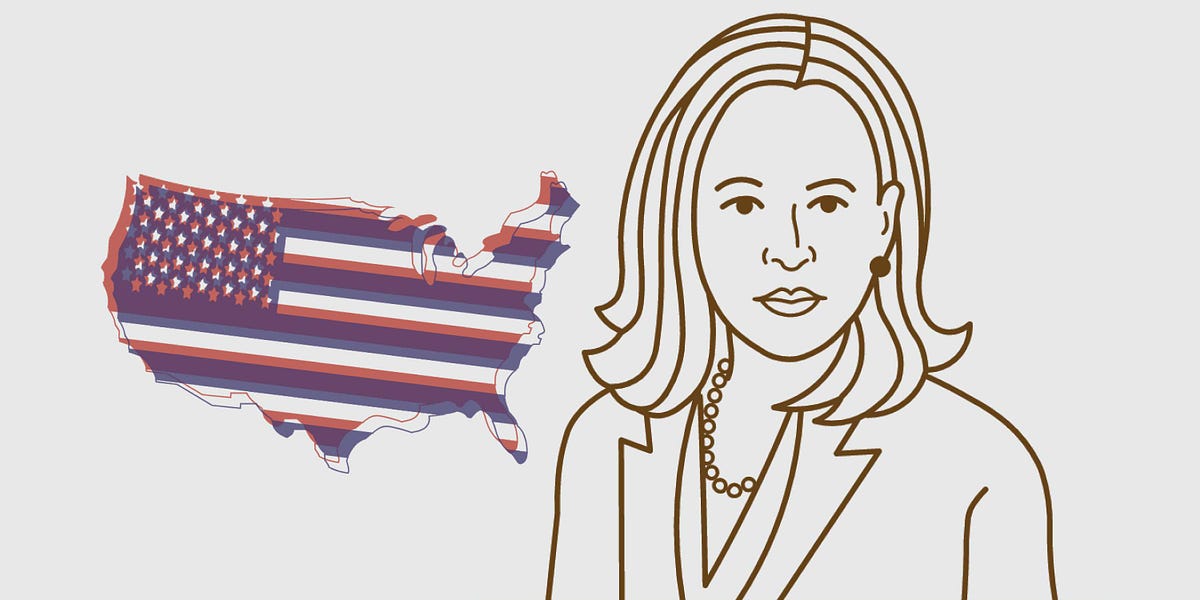The image is a computer-generated, cartoonish-style drawing featuring a woman and a graphic of the United States. The background is light gray, and the woman is depicted from the chest up, facing forward. She has shoulder-length, slightly wavy hair parted in the middle, and her features include full lips, open eyes, and a nose. She wears a circular earring and a pearl necklace, while her attire consists of a blazer or jacket. The woman is rendered in dark brown or black outlines.

To the left of the woman is a colored graphic of the United States, characterized by a glitchy effect. This graphic uses red, white, and blue layers, resembling newspaper print, with stars incorporated into the design, symbolizing the American flag. The combination of these elements creates a striking visual contrast between the detailed, monochromatic woman and the vibrant, layered U.S. graphic.